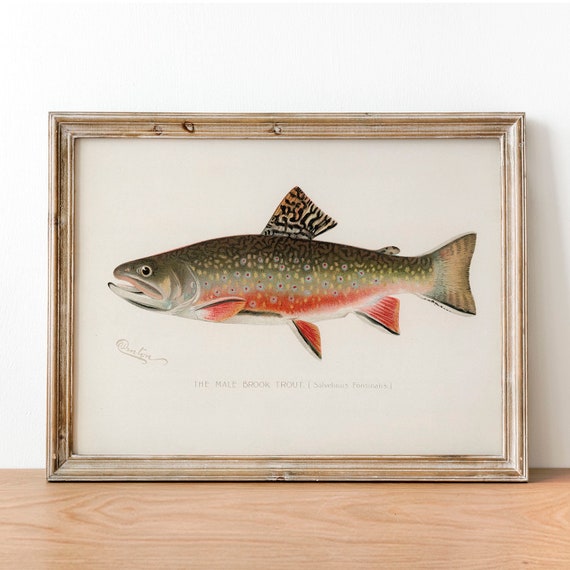The image presents a digital photograph of a painting with a fish as the central subject. Enclosed in a very basic, possibly vintage metallic bronze frame, the fish appears to be displayed on a nondescript pale wood grainy surface. The painting features a fish that is identified primarily by its distinct coloration: it has a reddish belly and an olive-green top adorned with gold speckles. The fish's mouth is open and facing to the left, giving it an alert and engaged appearance, while its eyes are wide open. Details include a bulbous side above the mouth, intricate black and red gill structures, and a short, tan and black tail. The fish has three fins on the bottom and one fin on the top. The background within the frame is a dirty white, and there is extremely faint text midway between the bottom edge of the painting and the fish. Overall, the image combines modern digital elements with a touch of vintage charm, highlighting the detailed and vivid depiction of the fish.